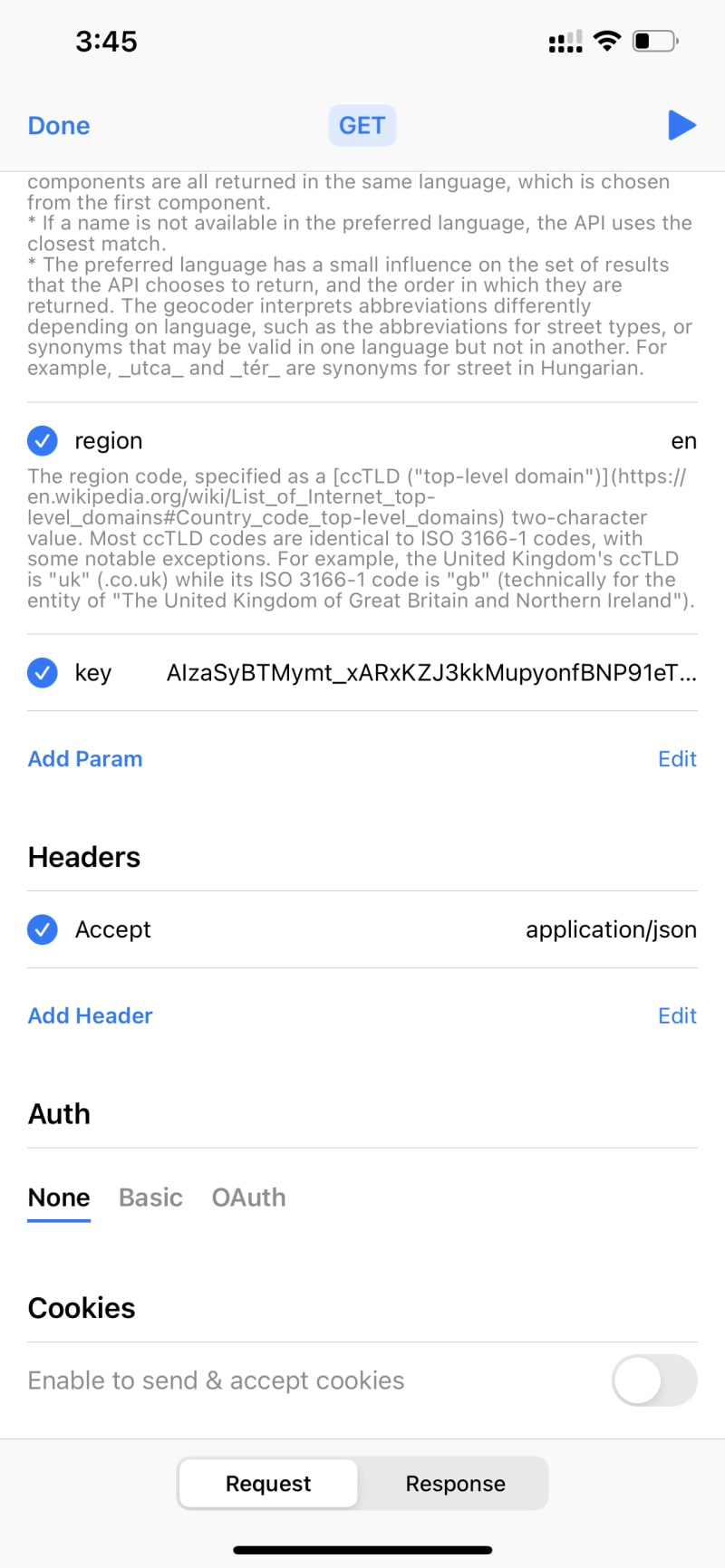The image displays a screenshot of a website interface, labeled as "345." At the top, there are two parallel lines and two bars, resembling signal strength indicators, where typically five would be shown. This is followed by an ellipsis ("..."). The Wi-Fi icon appears fully filled, indicating a strong connection. To the side, a progress bar is completely filled, and there is a "Done" button in blue text.

In the middle section, several gray squares are displayed, interspersed with clusters of blue squares forming an arrow shape pointing to the right. There is also a text snippet that reads, "Components are returned in the same language which is chosen from the first option. If a name is not available in the preferred language, the system uses the closest match. Your preferred language has a small influence on the set of results that the API returns and the order in which they are returned. The geocoder interprets abbreviations differently depending on the language. Some abbreviations may be valid in one language but not in another. For example, synonyms for 'street' vary."

Further down, the text continues with additional instructions, such as specifying the region with a region code and adding parameters to headers to accept applications. It also touches upon managing cookies and responding to requests.